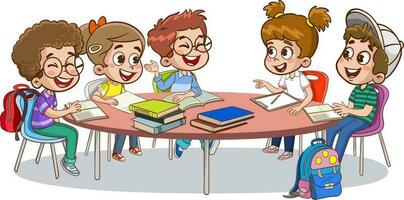This animated image shows five grade school children, joyfully engaging at a rounded brownish-colored table adorned with books, notepads, and clipboards, all set against a white background. Each child is vividly illustrated with open mouths, implying they are laughing and conversing excitedly. From left to right: a child with light brown hair and glasses wears a purple and green outfit, a girl with brown hair and a yellow and blue outfit sits next to him, followed by a boy with red hair and glasses dressed in blue shirt and pants. Next is a girl with brown hair in pigtails, clad in a white shirt and blue pants, and finally, a boy with brown hair under a white baseball cap, wearing a green striped shirt and blue jeans, seated near a blue and yellow backpack. The table casts a subtle oval shadow beneath it, emphasizing the lively and animated atmosphere, indicative of a fun, educational setting.